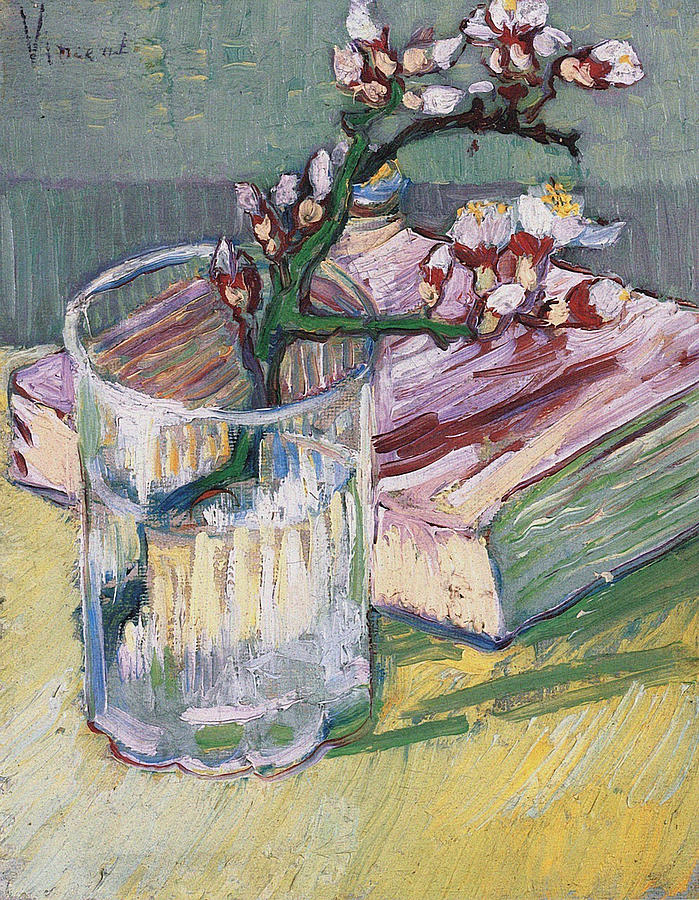The image is a detailed painting with a vertical rectangular orientation, signed at the top left though the name is indistinguishable beyond starting with a "V". Central to the composition is a clear glass jar serving as a vase, positioned slightly left of center and two-thirds filled with water. Emanating from the water is a flowering branch that extends upward and right-ward. At the top of the glass, the branch splits: one segment with a bud veering left and several other buds studding the rightward extension. Toward the top of the painting, the branch forks again with buds gracing the ends. These buds exhibit a palette of mostly white petals tinged with yellow and brownish-red bases. Adjacent to the glass is a book, distinguished by its vibrant pink cover. Its side and pages are tinted in shades of tan, purple, green, and white. The scene rests on a tabletop characterized by a yellow and white marbled appearance, with green streaks to the right of the glass. The background transitions from a purplish hue at the bottom to a gray-blue toward the top where the signature resides, marked by visible thick brush strokes, adding texture to the painting.